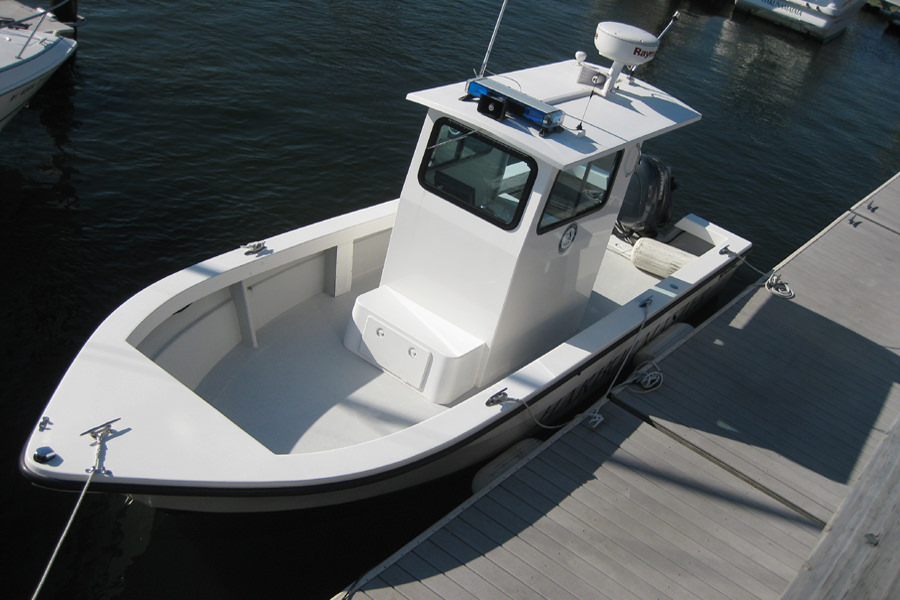This color photograph features an overhead view of a small white boat anchored at a wooden pier, which runs diagonally from the bottom to the right side of the image. The dark, calm water surrounding the boat ranges from a deep blue to nearly black. The boat, characterized by its sharp pointed bow and small size, can comfortably fit around ten people. At the center of the boat stands a semi-enclosed structure that resembles a small house or pilot's booth with windows on three sides, used for navigation and control. This structure is equipped with various antennas and a blue light on top. Additionally, there's a small black motor visible at the back of the boat. The background also hints at the presence of other boats, with partial views of them located at the top left and top right.